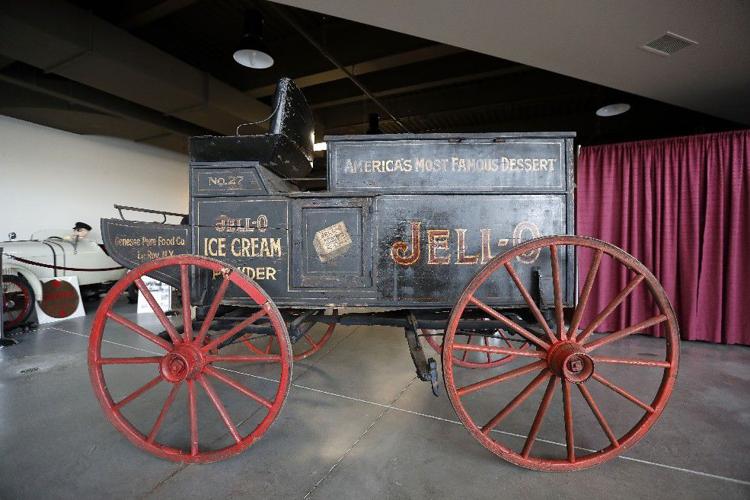The photograph depicts a historical wooden wagon set inside a warehouse. Dominating the foreground, the black wagon boasts giant red wheels and vivid gold text that reads "America's Most Famous Dessert" and "Jell-O," alongside "Number 27 Jell-O ice cream powder." The vehicle, likely a horse-drawn carriage designed for advertising and selling Jell-O products, features a distinctive black seat for the driver atop its square, suspended frame. The scene is anchored on a dark gray concrete floor marked with white lines. In the top left corner, an old white vehicle with red wheels and a red-and-brown circular sign is partially visible. Meanwhile, a maroon curtain and a heating air vent adorn the background, adding to the warehouse's nostalgic atmosphere.